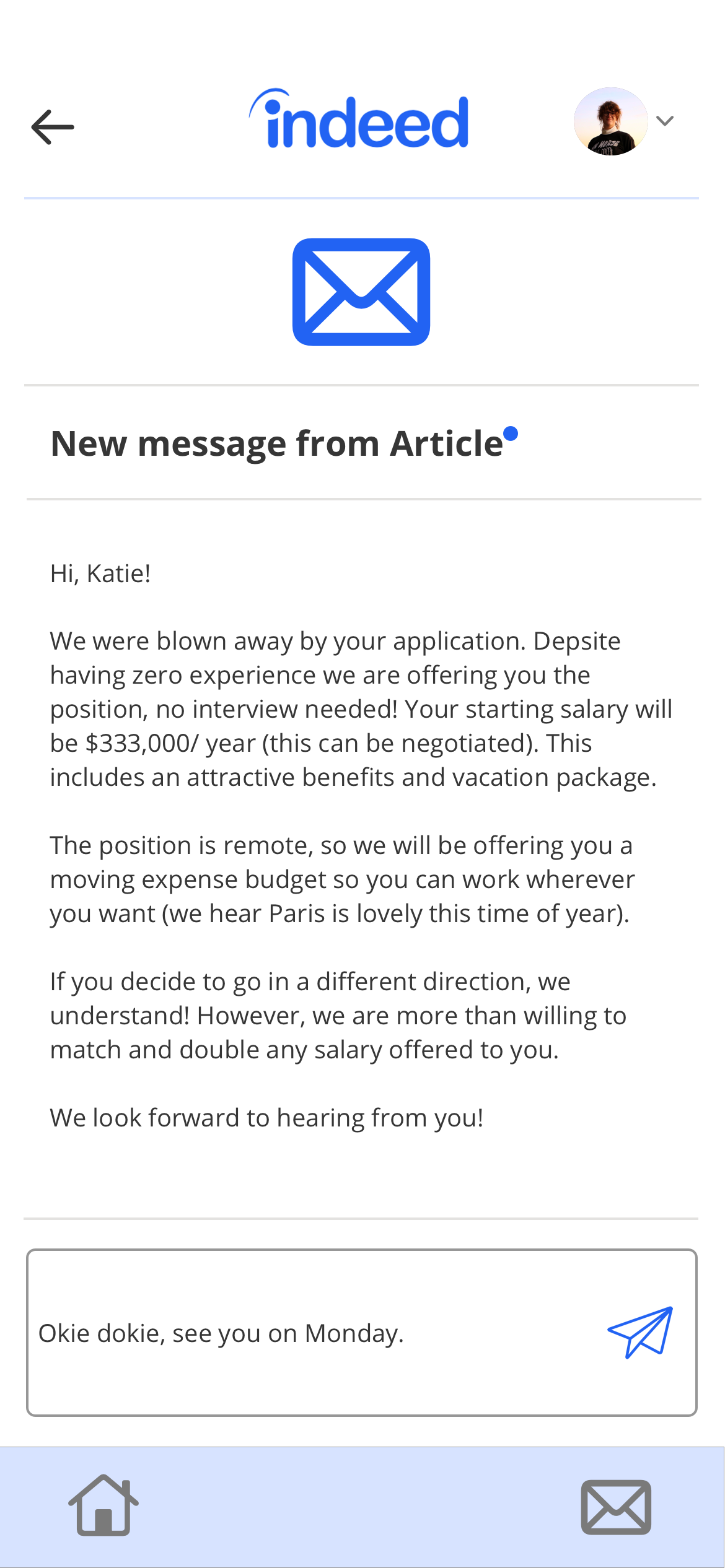The image showcases a humorous, fictional email notification on a white background. 

In the top left corner, a black arrow pointing to the left provides a navigation cue for "Go Back." Centrally placed is the "Indeed" logo, presented in a blue font signifying the job search company. To the right is a circular profile picture of a woman with black, curly hair, and wearing a black T-shirt. 

Next to her image, a small gray down-arrow is seen, leading to a gray horizontal line that divides the content. Below this line is a blue envelope icon, indicating a new message. The notification reads: "New message from article" with a blue dot symbolizing an unread message. The message begins with "Hi, Katie!," and continues in black text: "We're blown away by your application. Despite having zero experience, we're offering you the position, no interview needed! Your starting salary will be $330,000 per year. This can be negotiated. This includes an attractive benefits package. This position is remote, so we'll be offering you a moving expense budget so you can work wherever you want. We hear Paris is lovely this time of year. If you decide to go in a different direction, we understand! However, we are more than willing to match and double any salary offered to you. We look forward to hearing from you."

Below the message is a gray bar followed by a reply area. The applicant responded with "Okie dokie, see you one day." A blue paper airplane icon signifies the send button. 

At the bottom of the image, a gray navigation bar houses two icons - a house on the left and a mail envelope on the right, indicating home and mail options. The entire setup conveys a playful, satirical take on a job offer email, filled with exaggerated and unrealistic benefits.